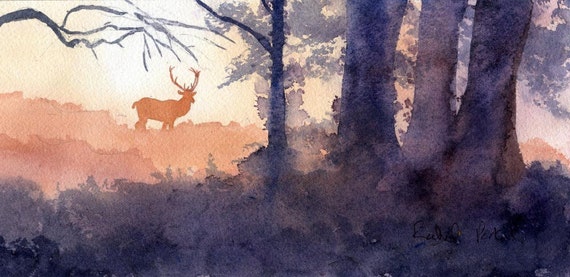The image is a vivid watercolor painting of a forest scene, set on a rectangular horizontal canvas in landscape mode. Dominated by deep blues and warm oranges, the artwork showcases a nighttime environment with intricate brush strokes. The foreground features three thick tree trunks on the right, painted in dark blue hues to signify the nocturnal setting. Central to this scene, a thinner tree stands out with a branch extending from the top left, draping towards the right. Below this canopy, a layer of light blue and brownish bushes adds complexity to the landscape. The heart of the painting, however, is an orange silhouette of a deer or buck, positioned center-left. This buck, with prominent antlers, stands as a striking contrast to the dark background, suggesting it is backlit by a yellowish-orange sky, adding a warm glow to the otherwise cool palette. The deer’s head is turned towards the viewer, and the silhouette, though sufficiently detailed, retains the painting's watercolor essence.